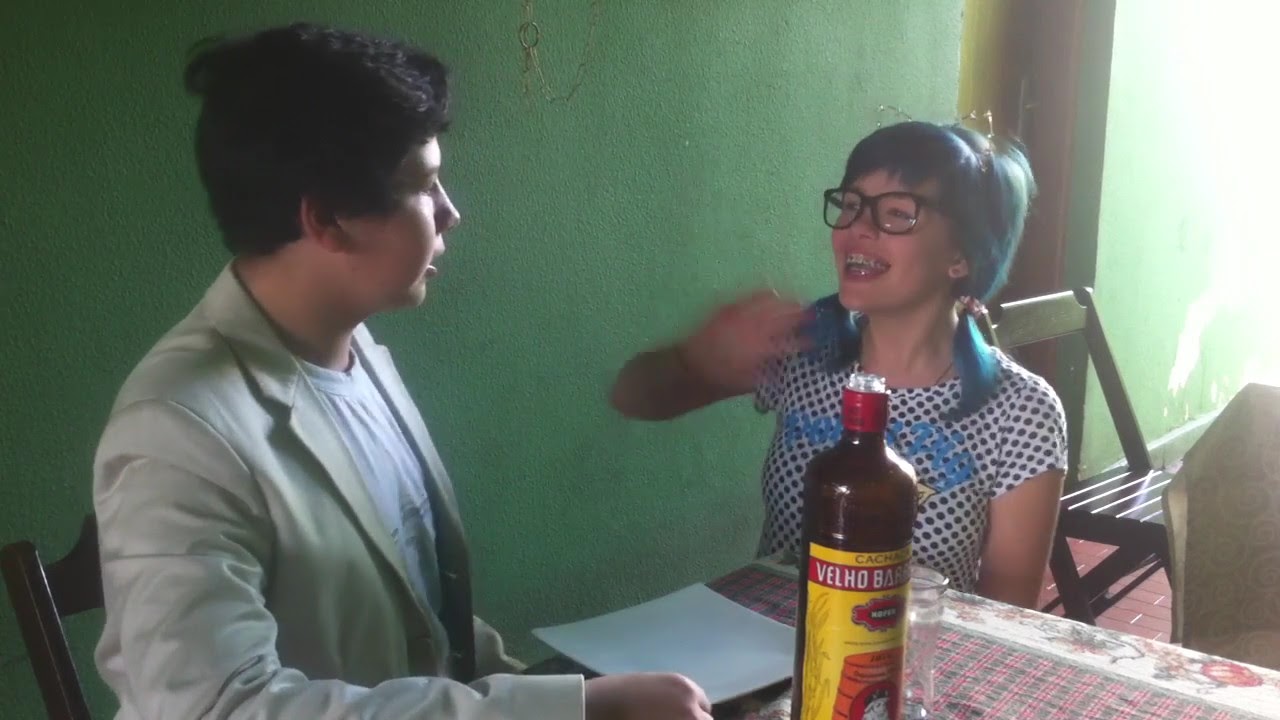In a cozy living room bathed in natural light from a nearby window, a young Asian man in his 30s is seated at a wooden table. He is dressed in a gray sport jacket over a white t-shirt and appears to be engaged in a lively conversation. In front of him rests a piece of paper and a brown bottle labeled "VELHO BAR C-A-C-H-A" hinting that it could be liquor. Opposite him sits a young woman with brown or black hair styled into two ponytails. She wears glasses and a checkered dress, and she is animatedly talking or smiling, her mouth wide open, and gesturing with her right hand. Behind her, a folding chair is visible, and the wall behind them is gray. The light streaming in creates a warm atmosphere, perfect for their engaging conversation.